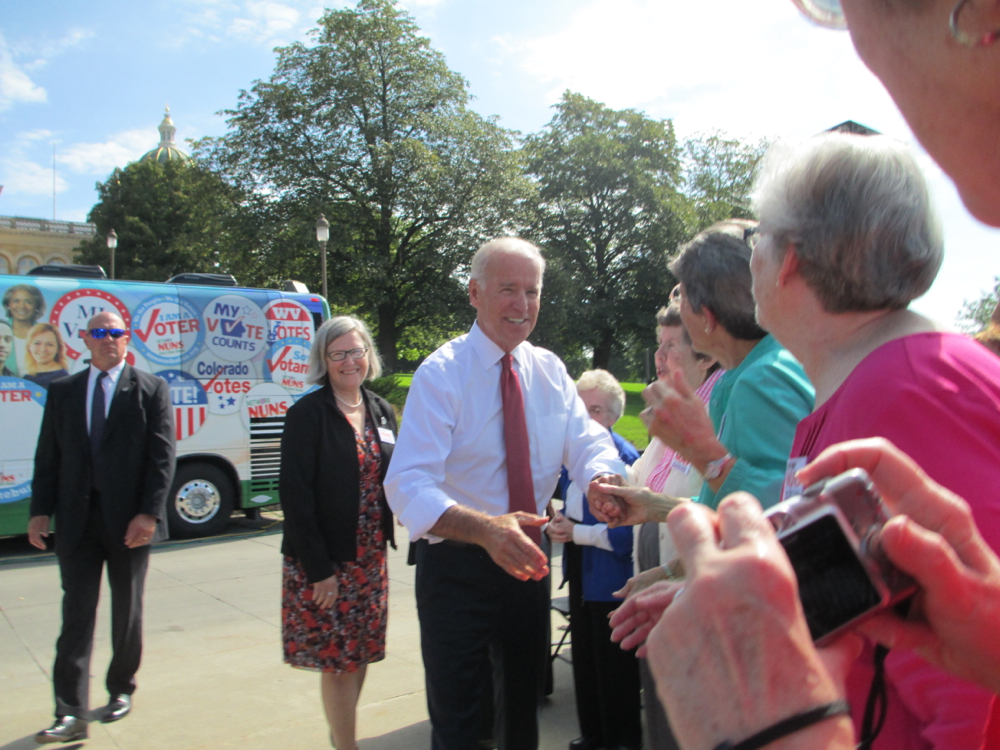The photo captures President Joe Biden meeting with supporters at an outdoor event. In the center of the image, President Biden, dressed in a white collared long-sleeve shirt with a red tie adorned with gray dots, and black pants, is warmly shaking hands with attendees. Notably, his sleeves are rolled up slightly, reflecting a casual, approachable demeanor. Directly interacting with him is a person in a green jacket. To his right, a woman in a pink long-sleeve shirt stands out, while several older women with short gray hair and turquoise sweater vests line up, eagerly awaiting their turn to greet the President.

Behind President Biden, a woman in a black sport coat and a black floral print dress featuring red roses and black spots watches over the proceedings, possibly his aide. An imposing man, likely a Secret Service agent, stands nearby, wearing a dark suit, a white shirt, a black tie, sunglasses, and black slacks. Partially visible on the left is another man holding a camera, with only his hands and part of his face in view.

The background showcases an atmosphere of camaraderie and anticipation, with a bus adorned with voter pins, green leafy trees, a blue sky with some clouds, and a partially visible bridge. The scene is set on a concrete sidewalk, emphasizing the outdoor aspect of this presidential interaction.